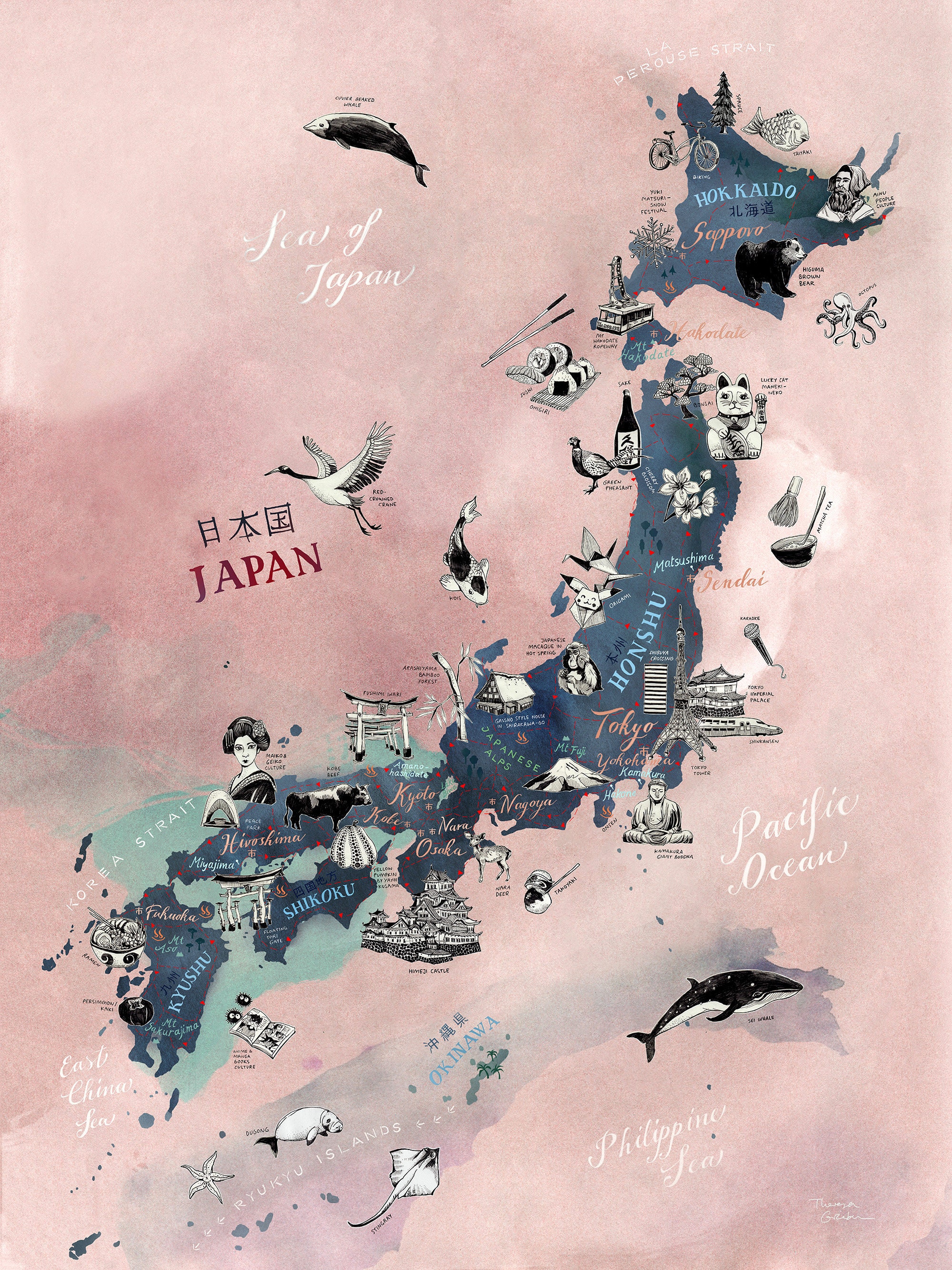This vertical, rectangular, multi-colored map of Japan is depicted in a heavily artistic and stylized manner with no borders. The background, where the water would be, showcases varying shades of pink with a watercolor effect, earning a sense of tranquility and delicacy. The main landmass of Japan stands prominently in a navy or greyish color, distinct against the soft pink background. Major regions like Hokkaido and Honshu are labeled in baby-blue hues, adding a bright contrast. Cultural and natural landmarks, such as temples, geishas, and diverse sea animals like whales, stingrays, and manatees, are depicted in black and white illustrations spread across the map. Smaller illustrations include a white crane, a bear, wine, and a Pikachu figure, highlighting regional specialties and cultural exports. The words "Japan" in red and Japanese script in black adorn the left side of the map, and the Pacific Ocean is labeled in white on the right. Notably, the map even includes smaller islands near Okinawa. This detailed and vibrant piece beautifully combines geographical information with cultural artistry.